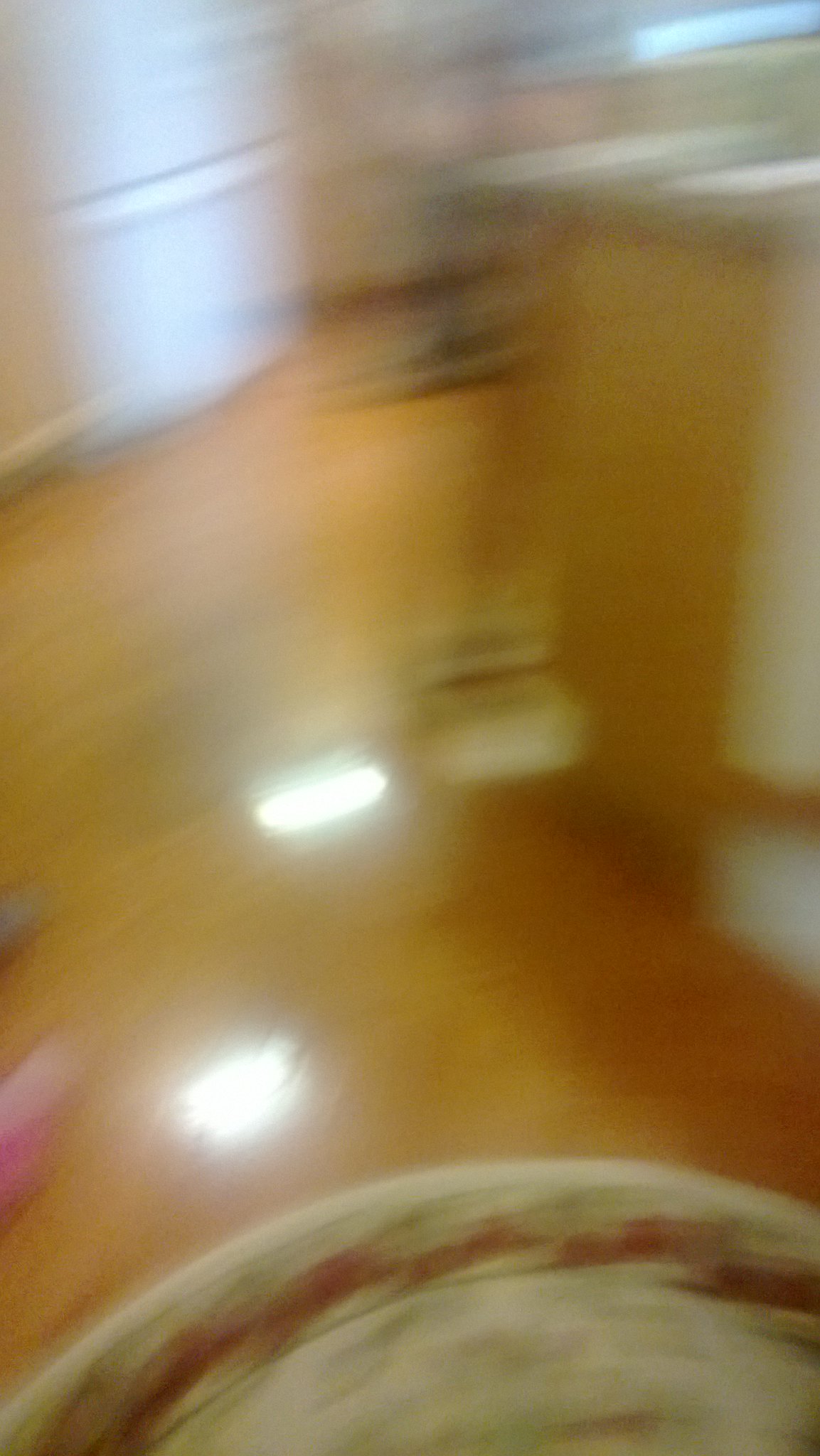This photograph, taken indoors, is notably blurred, obscuring fine details. However, discernible features include a light-colored wood floor that reflects the overhead kitchen light, adding a soft glow to the scene. In the upper left-hand corner, there appears to be a refrigerator with a dual-door design, having separate compartments for the top and bottom. To the right, a countertop is faintly visible, suggesting a typical kitchen layout. Although the image lacks clarity, the described elements hint at a cozy, functional kitchen space.